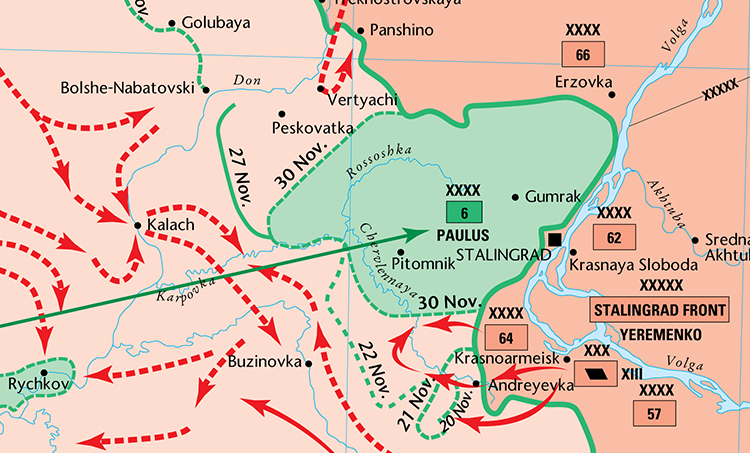The image depicts a detailed map of the Russian Empire during World War II, specifically focusing on the Battle of Stalingrad. Central to the map is the city of Stalingrad, marked prominently with an arrow and the label "Stalingrad Front." The map is vividly color-coded with pale orange and pale peach areas, and a smaller region highlighted in green. Numerous towns and cities are indicated by black dots, and the map includes intricate markings such as red and green arrows pointing in various directions, suggesting troop movements. Notable features include significant dates from November 20th to November 30th, red arrows indicating strategic advances, numbers denoting military units (62, 64, 57, 66) and symbols like X's, along with the names "Paulus" and "Volga River." The right side of the map, in a darker peach-reddish hue, appears to signify critical battle fronts and troop positions, highlighting the dynamic and chaotic engagements of the era.